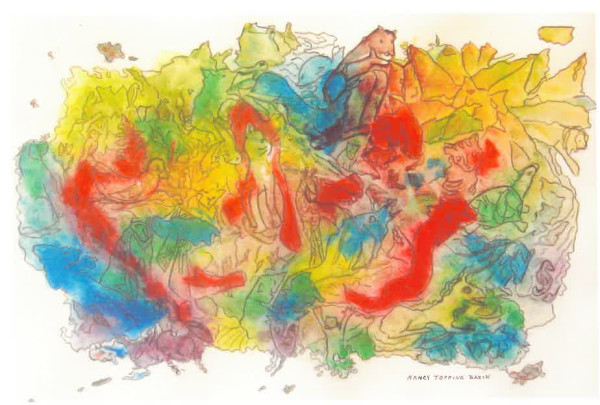The image is a horizontally oriented painting with a background that transitions from beige on the right to white on the left. The artwork features a dynamic, colorful compilation of various animals sketched in black silhouette and painted with splashes of vivid colors like red, blue, yellow, green, and beige. Crowded together in this imaginative piece, you can spot a bear at the top, a fish adjacent to it, a bird to the left, a cat, a turtle on the right, and possibly a horse. The animals are illustrated in a fragmented manner, resembling torn scraps of paper or leaves, blending together seamlessly. Towards the bottom, there is a blurry signature in gray letters, possibly reading "Nancy Topping," and the title "Basin." The painting is lively and intricate, capturing a whirlwind of wildlife in a uniquely stylized and compressed format.